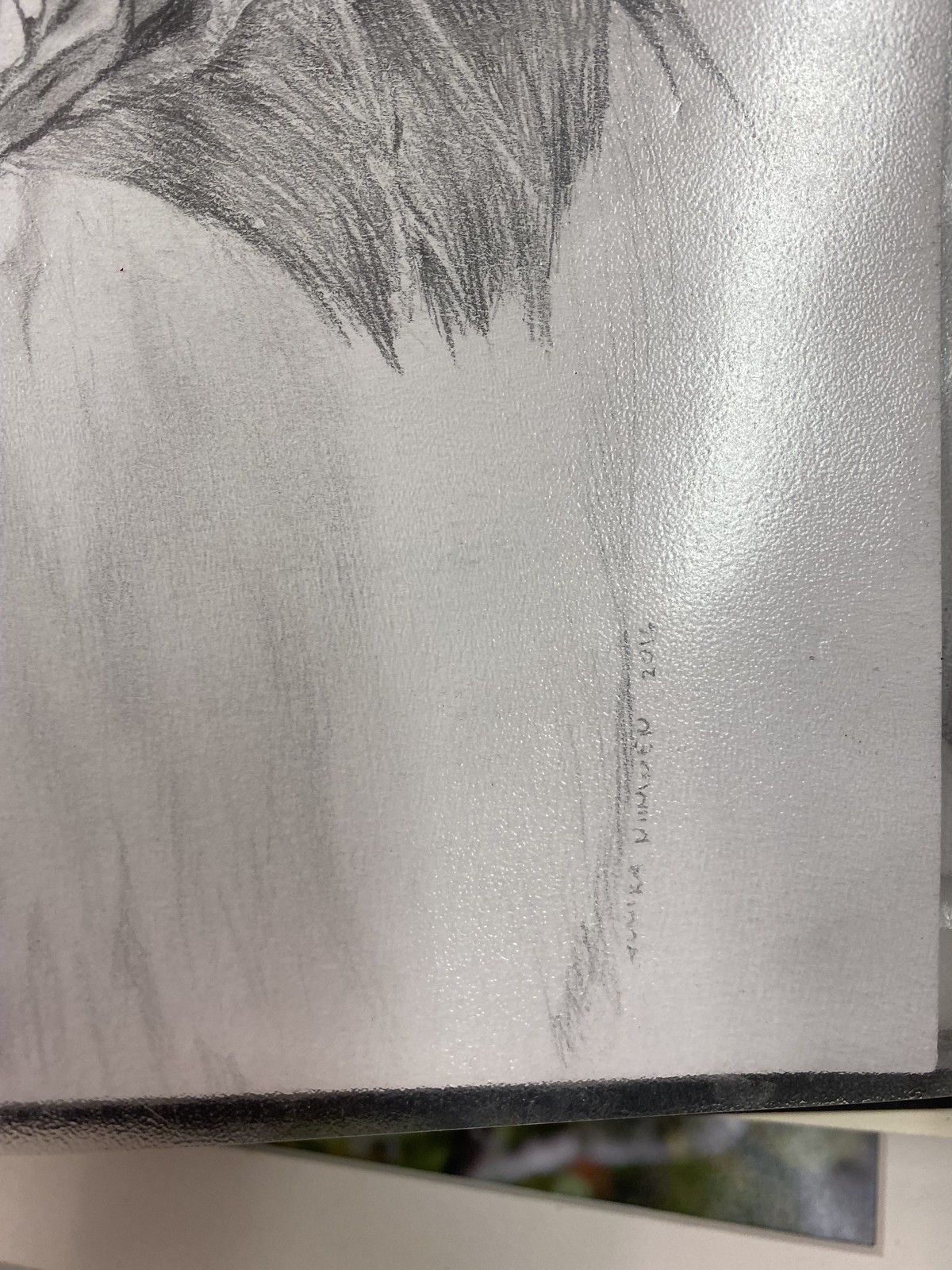This indoor color close-up photograph showcases the lower right corner of a pencil sketch resting on a shiny white surface, possibly a table. The sketch is encased in a black frame and features a discernible date of 2016 beside an illegible vertical signature, with speculative letters "N I M N E N." At the bottom of the photo, a strip of an off-white wall and a possible gray-toned, blurry window with trees are visible in the background. The upper left part of the drawing depicts a back view of a person's shoulder, faintly shaded with dark, straight hair cascading down. Light and dark pencil strokes create subtle shading throughout the sketch, with a notable glare reflecting from the upper right corner, adding a glossy impression to the artwork. The photo also hints at other prints lying underneath the featured sketch.